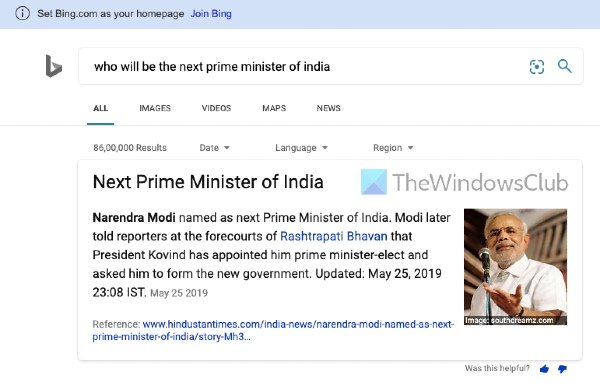The image is a screen capture of a Bing search page. At the top, there is a thin blue banner that prompts users to set Bing as their homepage, accompanied by a "Join Bing" button in blue. Below this, on the left, there's a gray Bing icon. The search bar contains the query, "Who will be the next prime minister of India?" alongside a blue camera icon and a blue magnifying glass icon. Beneath the search bar, there are navigation options labeled "All," "Images," "Video," "Maps," and "News," with a blue underline indicating the "All" category is selected.

The page then displays the number of search results and offers sorting options, including date, language, and region, each with drop-down arrows. The featured search result headline reads, "Next Prime Minister of India," followed by a snippet of the text: "Narendra Modi named as next prime minister of India. Modi later told reporters at the forecourts of Rashtrapati Bhavan that President Kovind has appointed him prime minister-elect and asked him to form the new government. Updated May 25, 2019, 23:08 IST." This text is accompanied by a reference in gray and a clickable blue link.

Adjacent to this text, there is a square banner in shades of blue, teal, and turquoise with the text "The Windows Club" in gray. Below the text snippet, there is an image of an older gentleman with light brown skin and gray hair, sporting facial hair. He is dressed in a white shirt and is positioned beside a microphone.